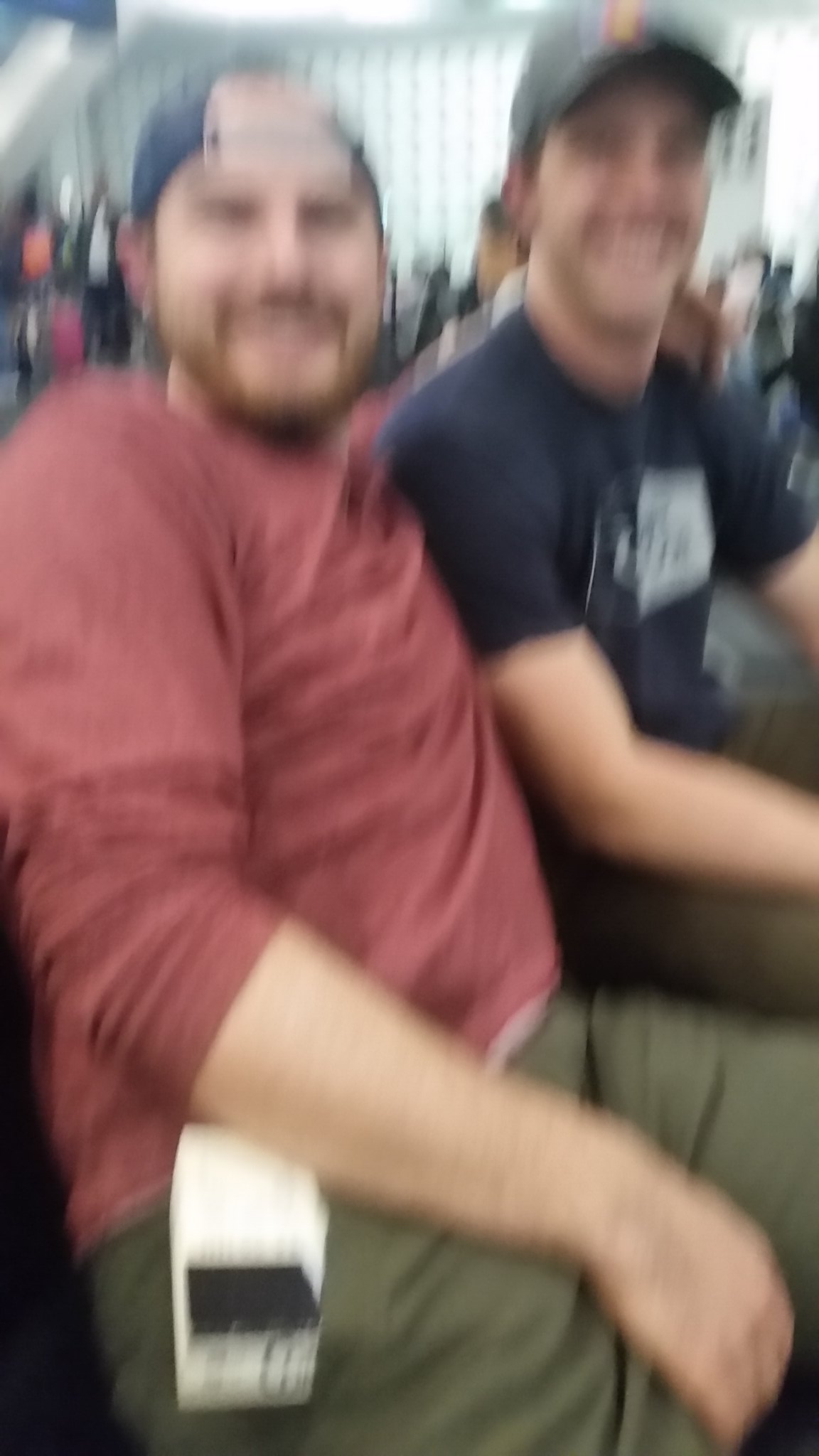In this photograph, captured in a candid moment, two friends are seen posing together. Despite the image being quite fuzzy and out of focus, certain details can still be discerned. The friend in the foreground, closest to the camera, is dressed in khaki pants and a dark salmon pink, faded red sweater. An object, either a piece of paper or an electronic device, is visible on his right hip. His right forearm is draped over his lap, and he is looking directly at the camera with a full beard of dark brown facial hair, an earring in his right ear, and a blue baseball cap worn backward. His left arm affectionately embraces his friend.

The second friend, sporting a wide smile, wears dark brown pants and a navy blue T-shirt with a white logo on the front. This friend has a clean-shaven face and is also wearing a blue baseball cap, this one oriented properly and adorned with a logo featuring yellow, red, and blue colors. Both friends are looking and smiling towards the camera to their right.

In the background, numerous people can be seen standing around, and further back, large glass windows are visible, suggesting this location might be an airport. The scene evokes a sense of excitement and happiness, possibly hinting that the friends are either awaiting a flight or are being seen off before embarking on a journey.